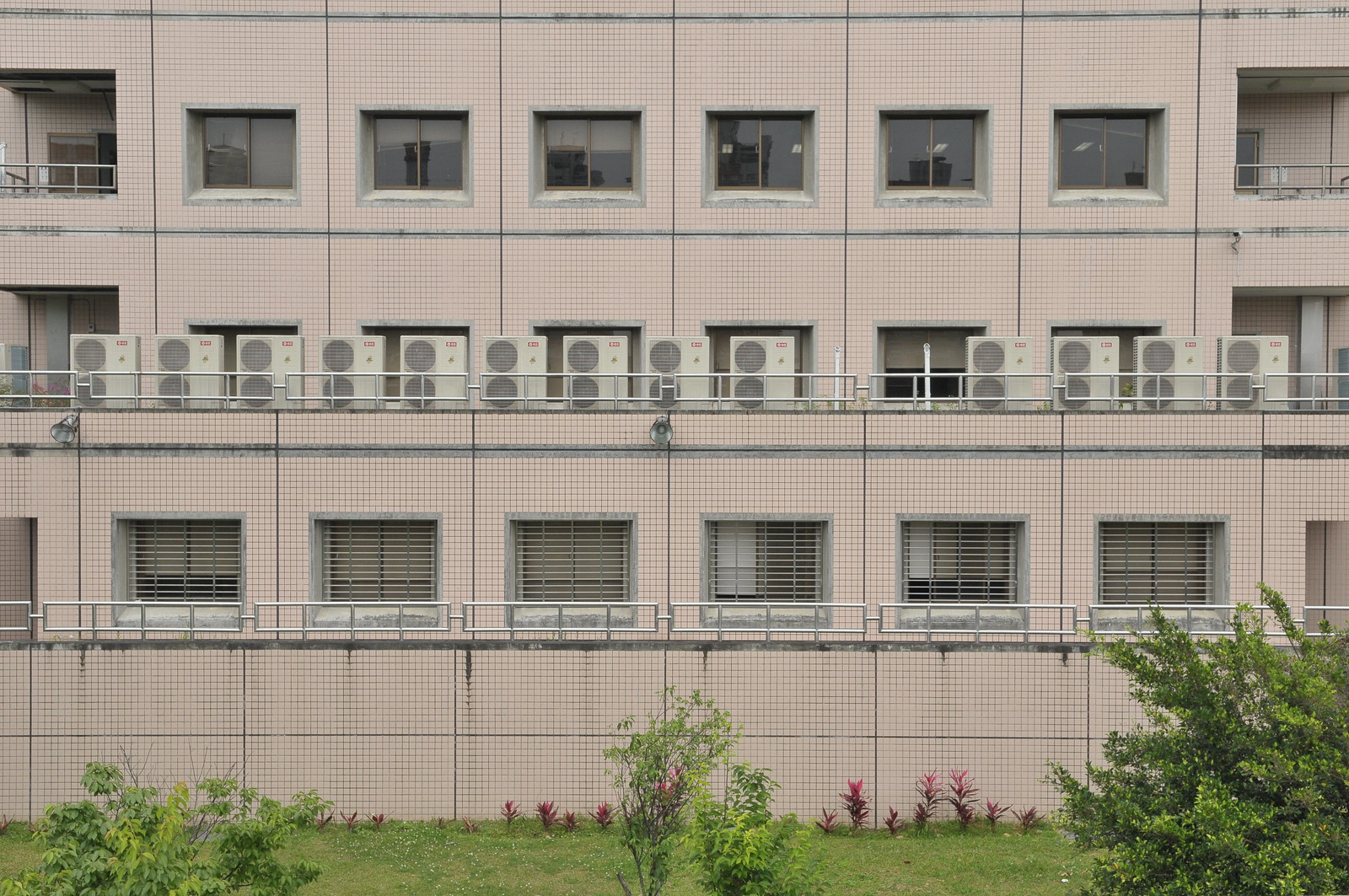The photograph captures the exterior of a three-storey apartment complex bathed in clear, neutral daylight. The building walls feature a light pink, almost off-white tone with a tiled pattern. Prominent balconies, lined with narrow railings, run across each level, contributing to a sense of symmetry and structure.

In the foreground, a vibrant green lawn stretches out, sprinkled with occasional patches of yellow. Nestled up against the building are striking red plants with leaves flourishing at various heights. Among them, three or four bushes of distinct sizes and densities are arranged: the largest and bushiest occupies the right, while the centre and left bushes are narrower and lighter in color.

The first two levels of the building's balconies are adorned with numerous air conditioning units. These units, identifiable by their white metal containers and dual round ports with grill-like features, hint at the cooling apparatus within. The third-floor windows are protected by metal guards, adding an extra layer of security absent from the lower floors.

Overall, this well-lit scene clearly articulates the aesthetic and functional aspects of the apartment complex, highlighting its greenery, structural details, and utilitarian elements.